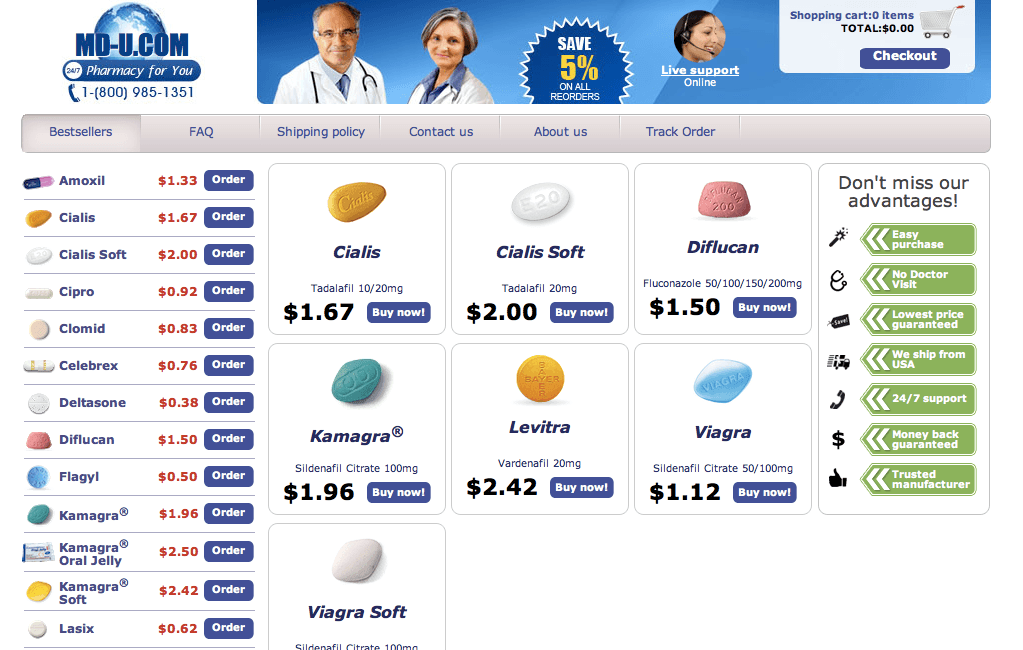Certainly! Here’s a cleaned-up and detailed descriptive caption for the screenshot of the website:

---

**Website Screenshot Description for md-u.com (Farms4U)**

The screenshot shows the homepage of the website md-u.com, also known as Farms4U. In the upper left-hand corner, a logo featuring a planet is prominently displayed. The top section of the page showcases a banner with an image of an older female doctor wearing a lab coat, accompanied by a small icon indicating live support—a pair of headphones—suggesting customer service availability. Additionally, there is a shopping cart icon located in the upper right-hand corner, which is currently empty.

A noticeable phone number, 1-800-985-1351, is present, providing a direct contact option for customers. Below the banner, the main navigation menu contains several options written in blue text on gray tabs. These tabs include: Best Sellers, FAQ, Shipping Policy, Contact Us, About Us, and Track Order.

The main content area lists various medications alongside their respective prices, such as Cialis for $1.57, Letbria for $2.42, and Viagra for $1.12. The focus seems to be primarily on sexual health medications. 

On the right side of the webpage, there is a menu titled "Don't Miss Advantages." This section features green bars with white text that highlight various benefits of shopping with Farms4U, such as "Easy Purchase," "No Doctor Visit," "Most Price Guaranteed," "We Help Ship from USA," "24-7 Support," "Money Back Guaranteed," and "Trusted Manufacturer."

Additionally, the left side of the page lists more medications, indicating that the website offers a variety of drugs beyond just sexual health products.

---